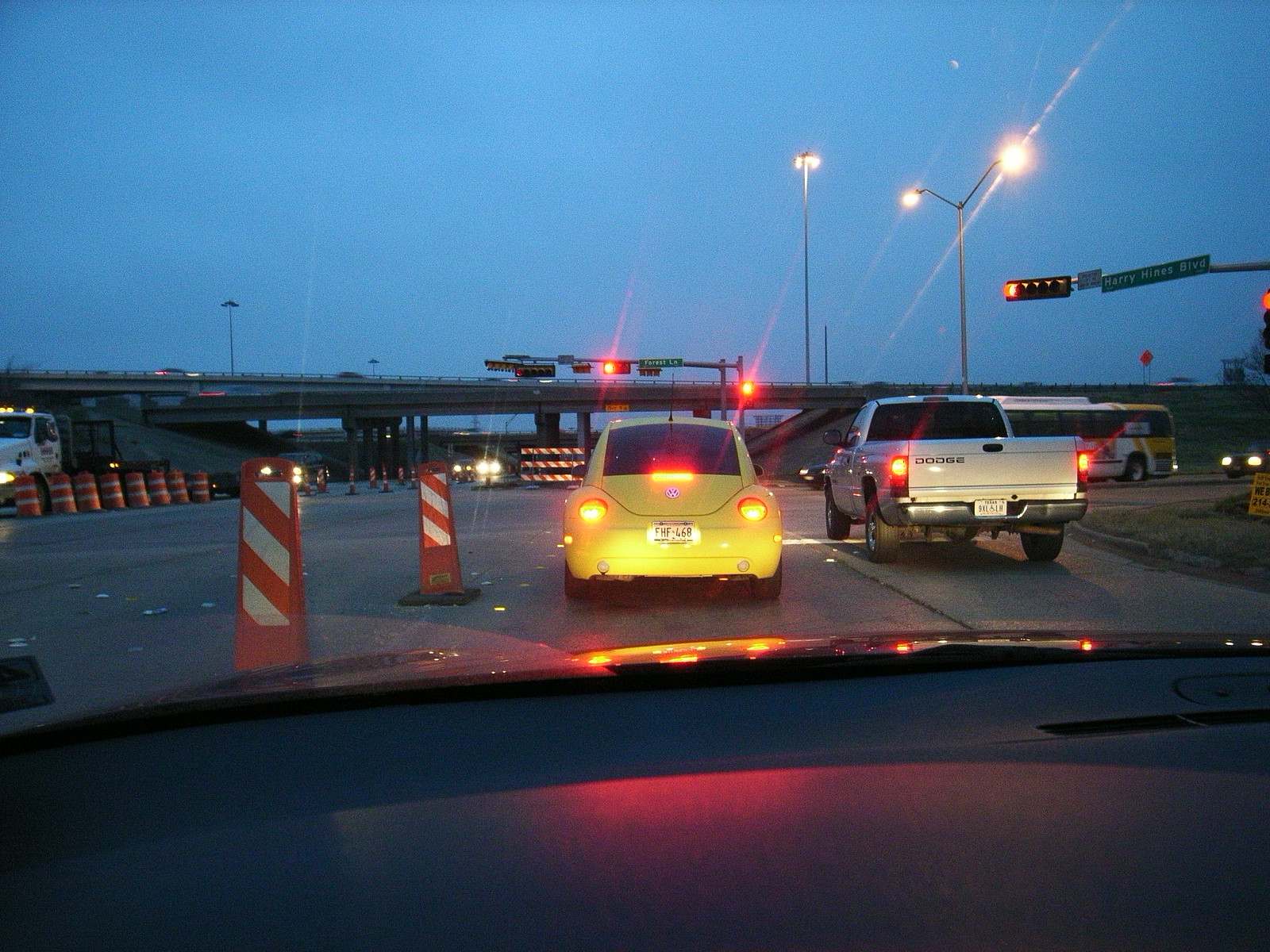This photograph, taken from within a vehicle, provides a dynamic view through the windshield, featuring the car's front hood prominently. Directly ahead, a yellow Volkswagen Bug with illuminated taillights catches the eye, while to its side, a white pickup truck is visible. Over these vehicles looms a white concrete overpass, adding an urban element to the scene. The street below is visibly rough and dotted with orange and white construction cones, indicative of ongoing roadwork. Streetlights, already lit, hint at either early morning or dusk. A red traffic light, mounted on a metal pole, commands attention in one corner of the image. Adjacent to the traffic light, a green street sign with white lettering provides location context. Additionally, a bus and another car are seen further behind, contributing to the bustle of the depicted roadway.